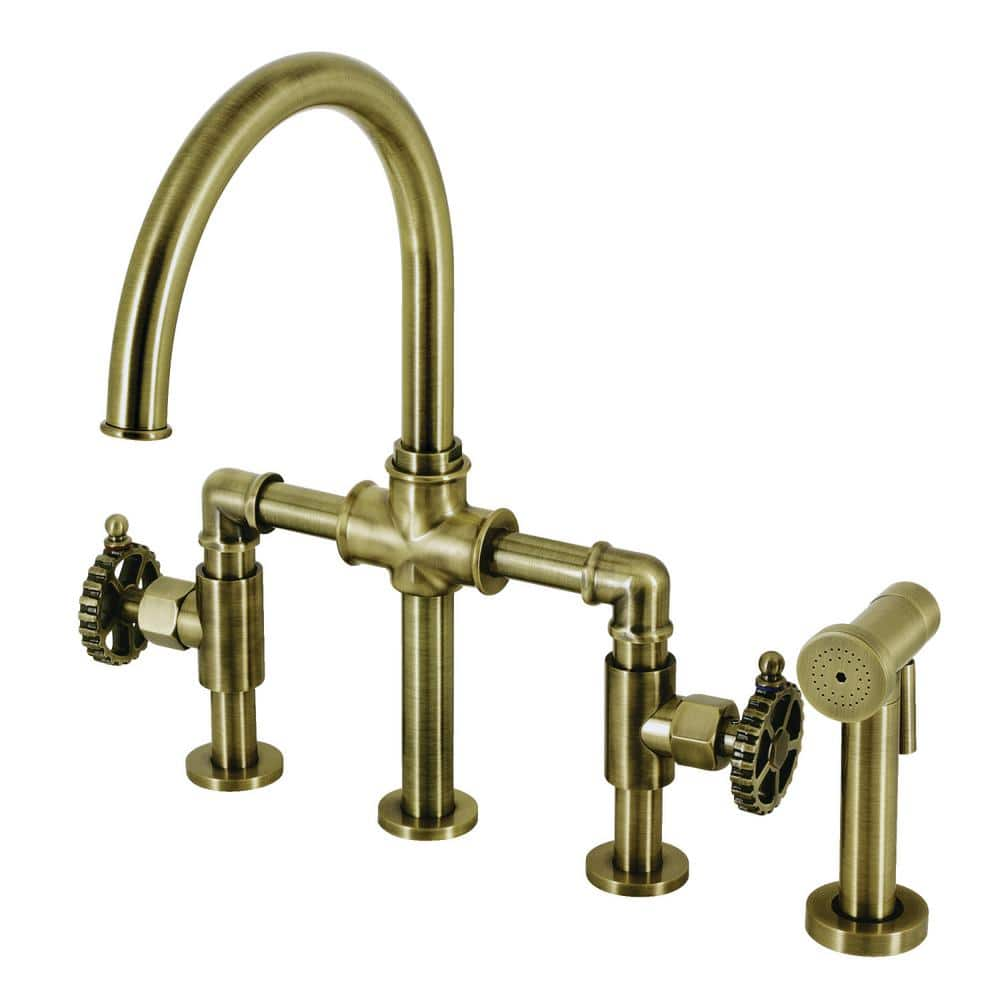The image depicts a steampunk-inspired kitchen faucet assembly against a completely white background, featuring detailed bronze-colored components. The centerpiece is a tall, curved spout flanked by two pipes that converge at its base. Each pipe is fitted with textured, circular gear handles for water control. Adjacent to the main spout is a matching bronze kitchen sprayer nozzle. The faucet and sprayer appear unfinished and unattached to any sink, resting instead on three supporting prongs. The overall aesthetic highlights exposed inner workings and gears, enhancing the mechanical, steampunk vibe of the design.